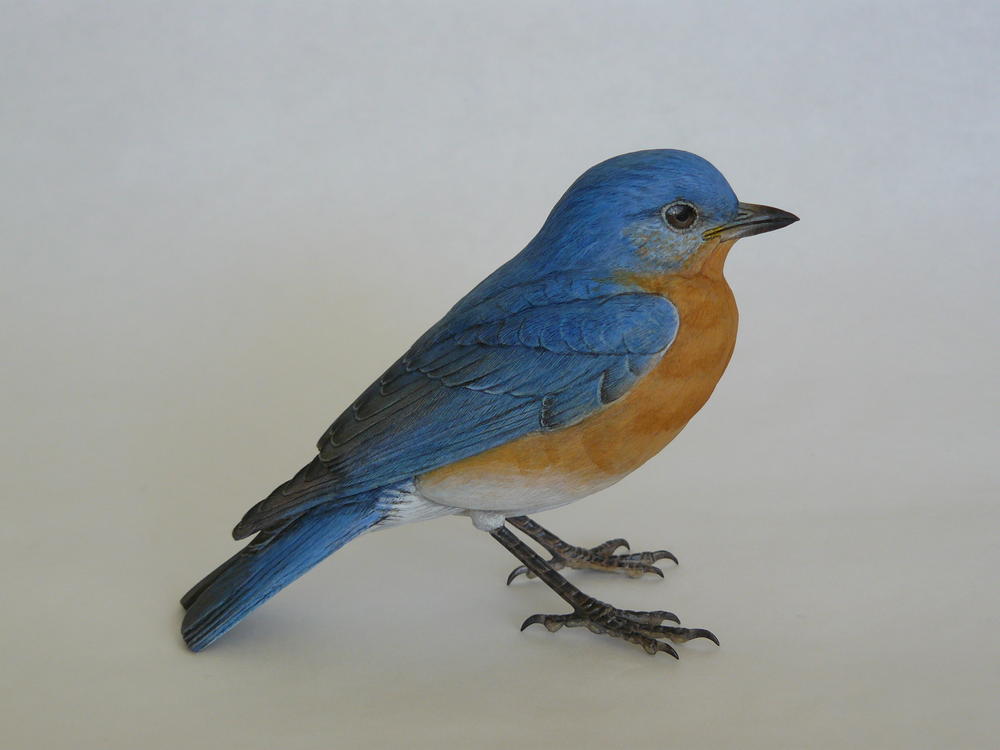This hand-drawn illustration showcases a small, round bird that could be either a blue robin or a tit, positioned against a seamless, neutral grey background that gives the illusion of the bird standing on an indistinct surface. The bird features a short, pointed, and dark beak along with striking brown eyes with dark irises. Its head, back, and tail are adorned with royal blue feathers, while the ends and tips of its wings and tail have a slight greyish tint. The chest of the bird is a blend of orange and camel colors, transitioning to white just above where its dark, clawed legs attach. The bird's legs, depicted with long phalanxes, display four claws—three facing forward and one pointing backward—suggesting it is poised and alert, perhaps having just spotted a worm or two for its morning meal.